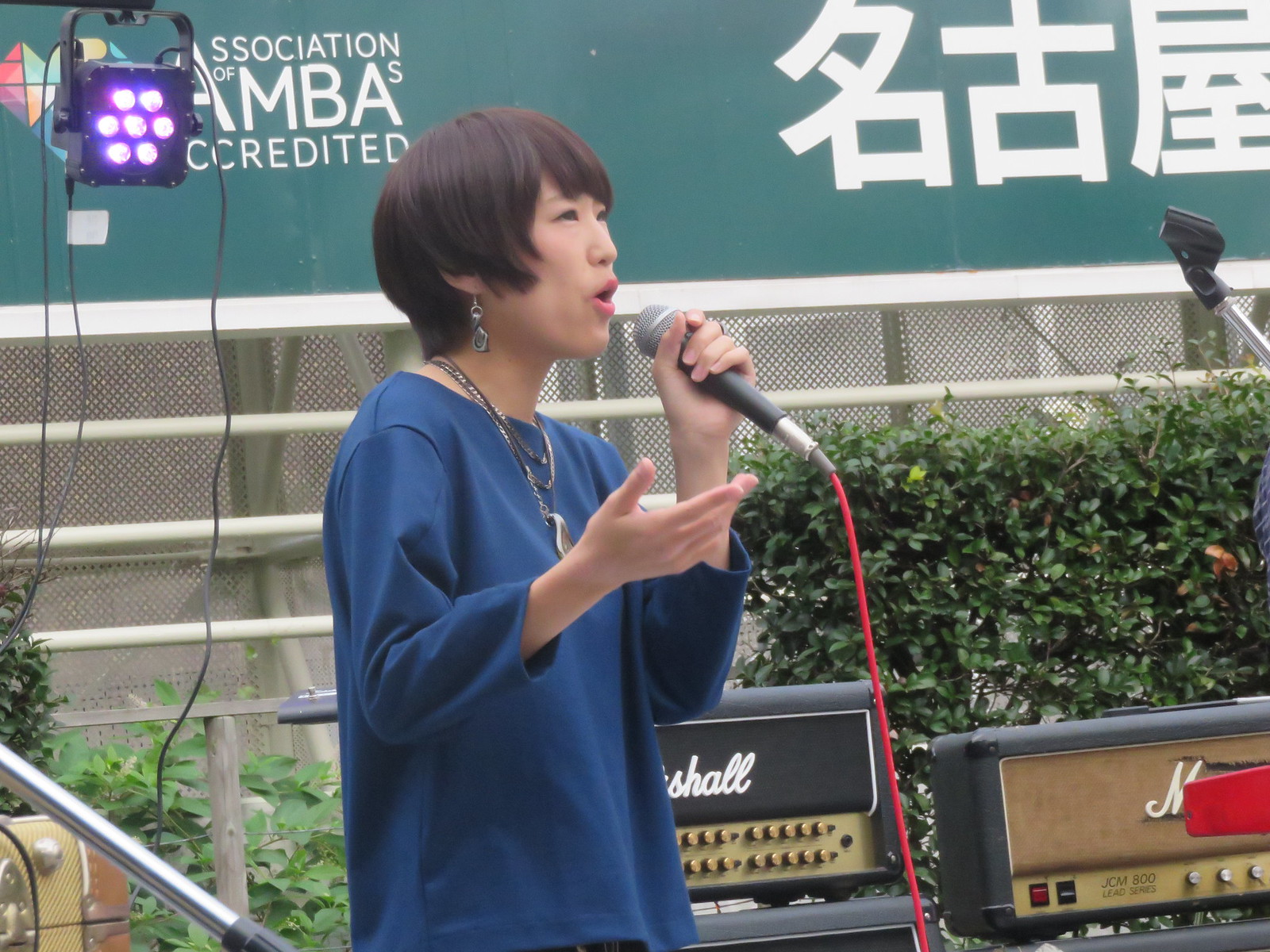In this lively outdoor photograph, a young Asian woman with a short, brown pixie haircut is captured mid-performance, holding a black microphone with an orange cord. She is adorned with earrings and necklaces, and dons a long-sleeved blue shirt. Her expressive stance, with one hand gripping the microphone and the other extended, suggests she's deeply engaged with her audience. The sunny daylight enhances the vibrant scene, which features a purple spotlight and a black case aimed towards the performer from the background. She stands confidently on stage in front of two large black Marshall amplifiers, which are brimming with buttons. Behind her, green shrubs and a fenced area are visible, along with a green and white sign that reads "Association, Accredited, MBAs," partially obscured by the spotlight. Above the sign, there are symbols of Chinese lettering, indicating that the event is related to a Chinese-speaking community. This image vividly depicts a moment at a conference or convention, highlighting the woman's dynamic presence against a backdrop of musical and cultural elements.